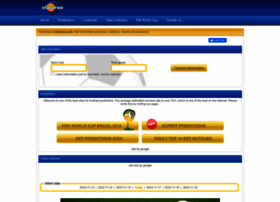This image appears to be a low-quality screenshot from a website, predominantly displaying a white background. At the top, a dark blue banner spans across, featuring an orange circle and white symbol within it on the left side. Directly beneath this, a lighter blue section contains white text, though it's too pixelated to decipher.

Below the light blue section is a narrow horizontal banner in yellow, followed by a small blue button or banner. Continuing down, there's a slightly wider blue separator. The next portion of the screenshot showcases several text boxes bordered in yellow, accompanied by a yellow button to the right. Another blue separator follows. Subsequently, four yellow buttons are aligned in a row.

Towards the bottom, another blue separator precedes a section where text is enclosed by a yellow border. The white background of the image includes a faint drawing, possibly a person with gray hair, but the low resolution makes it difficult to identify the specifics. The arrangement and color scheme suggest a structured design layout, likely intended for navigational or interactive purposes on the website.